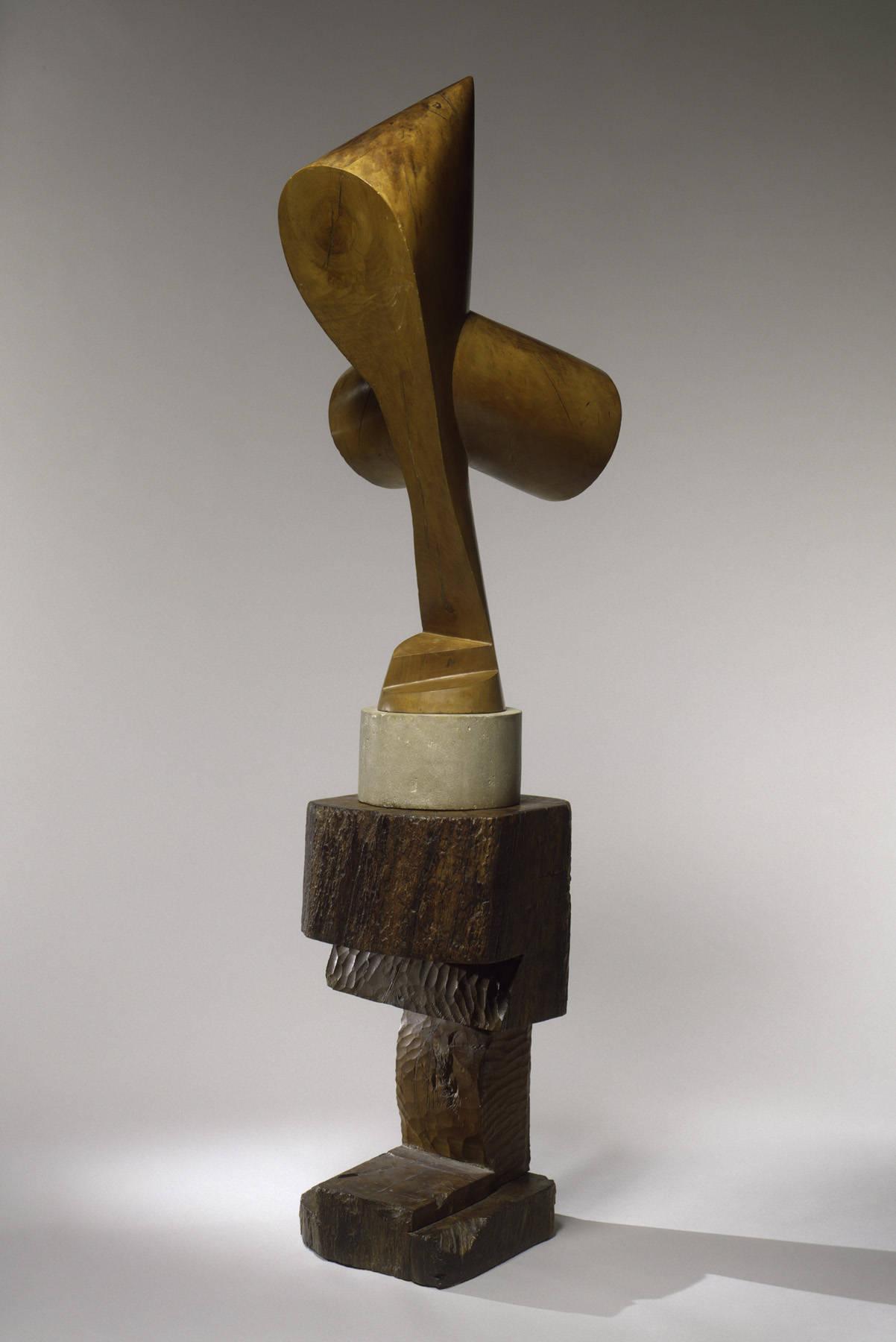The image features a fascinating abstract sculpture prominently centered within a rectangular frame. The backdrop transitions from a light gray at the bottom to progressively darker shades of gray towards the top, providing a subtle gradient that emphasizes the sculpture. The base of the sculpture is crafted from dark brown wood, intricately carved to resemble the letter "E" lacking its middle bar, with subtle indentations that suggest hand-carving. Atop this wooden base rests a cylindrical component, possibly made of marble, in a light gray or white hue. This cylindrical piece acts as a pedestal for the upper section of the sculpture. The top portion consists of an eclectic assortment of wooden elements. A dominant feature is a thick cross-like structure with one end resembling an oblong hammer, tapering to a point, and the opposite end extending into an elbow-like curve reminiscent of a PVC elbow, but sculpted from the same wood. The wood here varies in color from light to dark tones, further enhancing the composition’s intriguing, abstract nature.